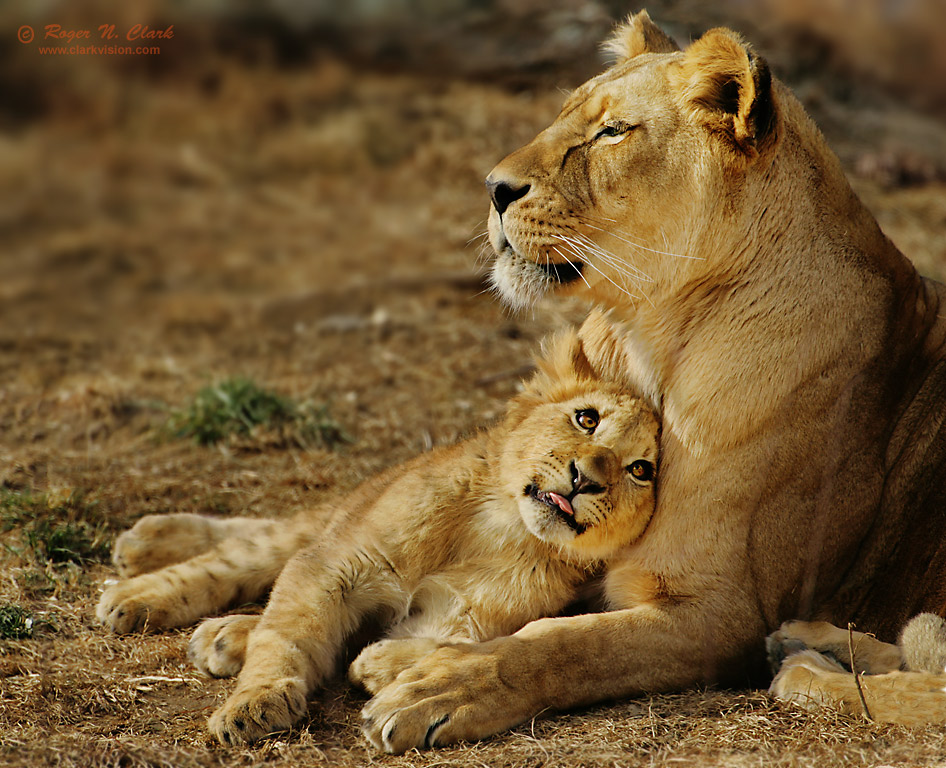In this striking digital photograph, a majestic lioness is captured in a close-up shot, exuding a stoic grace as she gazes to the left while reclining on a patch of dried brown savanna grass, interspersed with occasional green patches. Her golden fur radiates in the soft light, and her paws are stretched out in front of her. Nestled securely against her chest is a tiny lion cub, whose golden coat mirrors that of the mother. The cub’s orange eyes look up adorably at the lioness, with its little pink tongue peeking out slightly. The overall background is artistically blurred, highlighting the tender moment between the lions, and adding to the serene ambiance of the scene. The professionalism of this photograph is further marked by the top left corner text in red, reading "Roger M. Clark, Clarkvision.com, copyright."